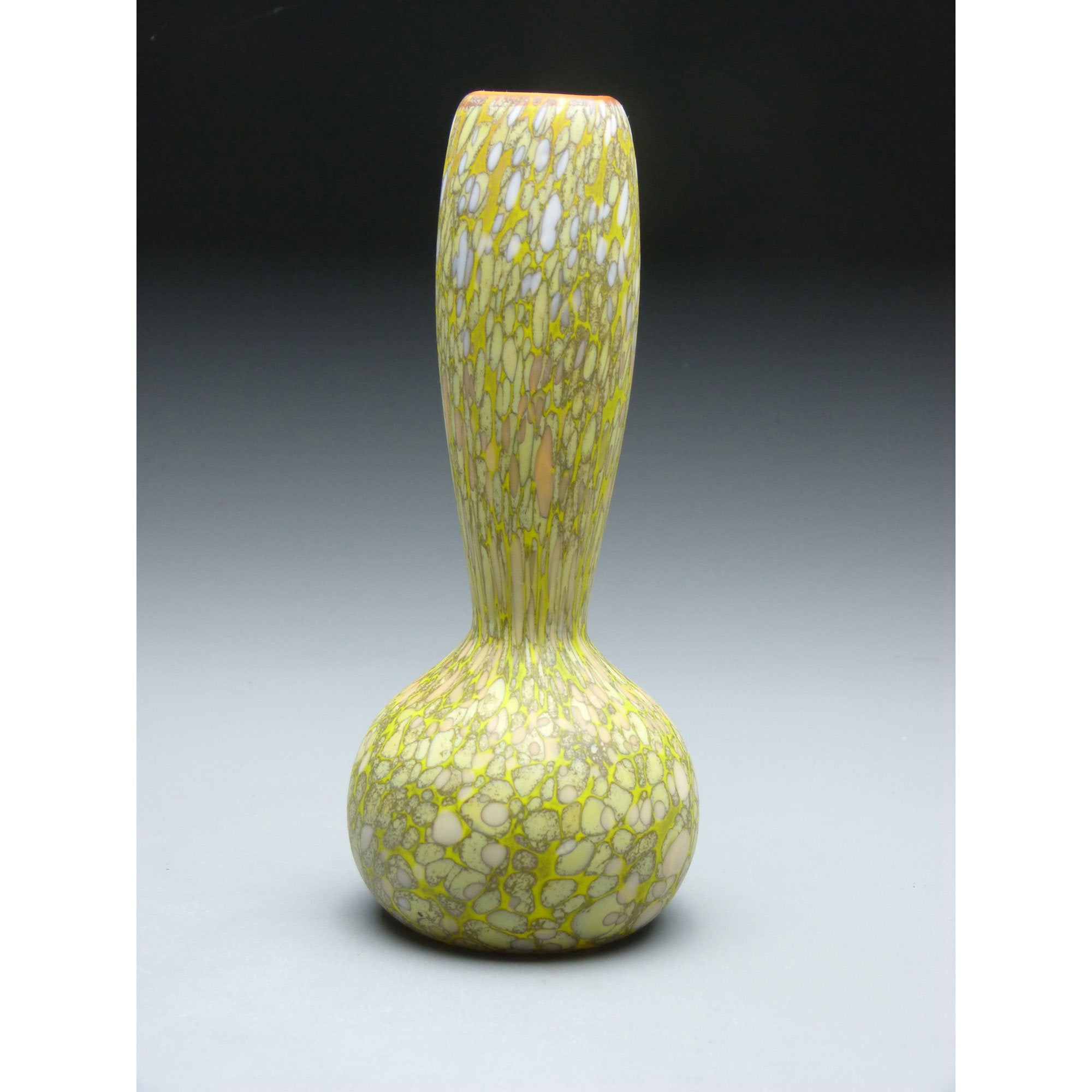This full-color, vertically rectangular photograph, taken indoors under artificial lighting, features a meticulously staged art object at its center. Set against a gradated background that transitions from black at the top, through gray in the middle, to almost white at the bottom, the object stands out vividly. The item, resembling a vase or gourd, boasts a round base with a flat bottom, ensuring stability. As it extends upward, the structure narrows significantly before widening again toward the top, culminating in a long, cylindrical neck that's longer than the base itself. The object is predominantly lime green, adorned with various white, yellow, and reddish shapes that resemble oval or gemstone-like patterns. Some spots on the object also appear green or light brown, adding depth and texture to its ancient, calabash-like design. The shadow beneath the vase further emphasizes the object’s three-dimensionality, while the overall composition suggests a purposefulness and artistic intent in the presentation.